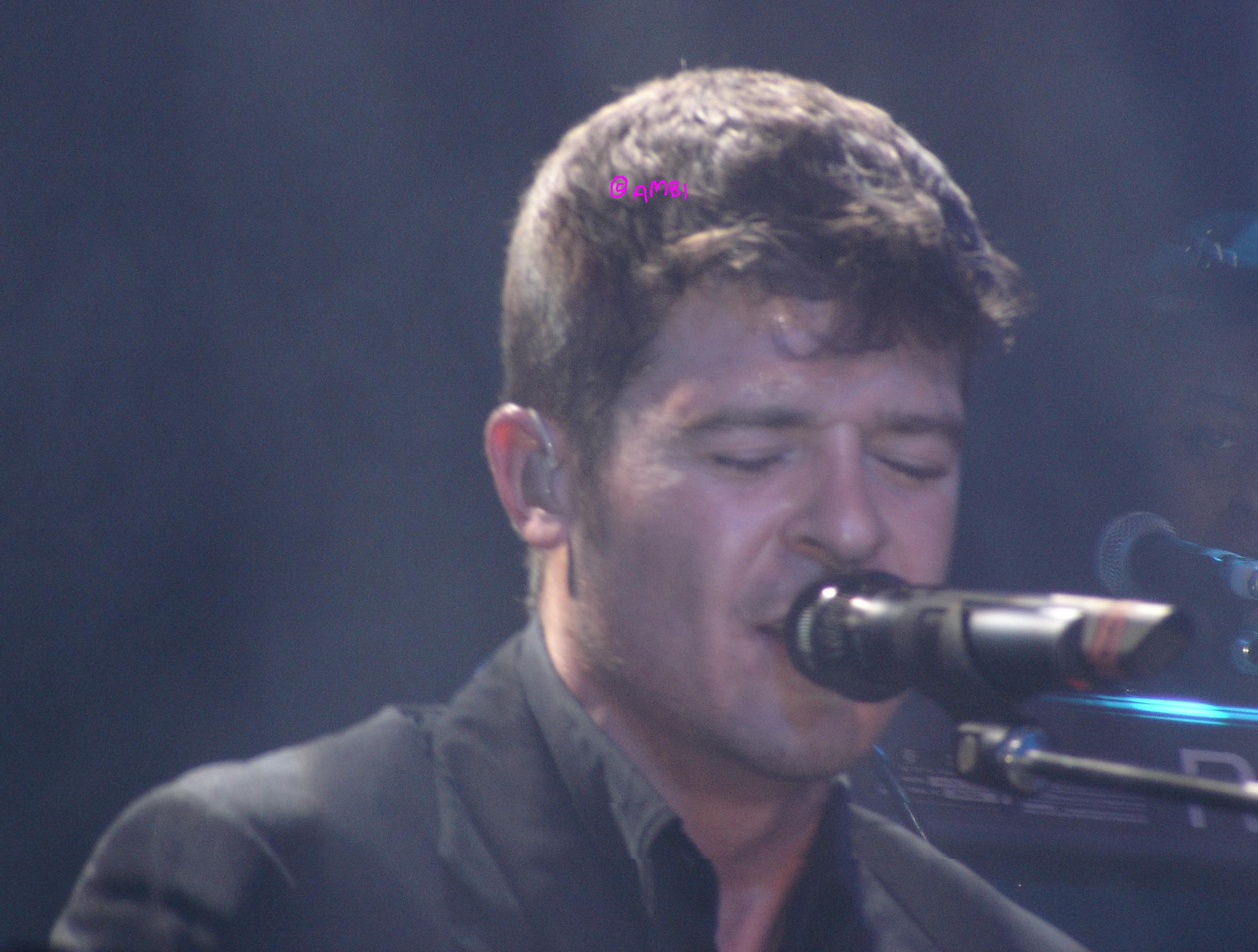The image is a very close-up photograph of a middle-aged singer performing passionately on stage. He has dark brown hair that peaks and curls over his forehead and is clean-shaven. His eyes are closed as he sings, indicating he is deeply immersed in his performance. A black wireless microphone is positioned close to his mouth, projecting his vocals. He wears a black suit jacket with an open collar, revealing the bottom of his neck. An earpiece is visible in his left ear, possibly for receiving communications from his team. The background is dark and smoky, with a magenta-colored font around his hair spelling out "AMBI" in all capital letters, which appears to be a social media handle. To the right side of the image, another face, likely a band member, is partially visible with a microphone in front of them. The setting suggests it is taken at a concert.